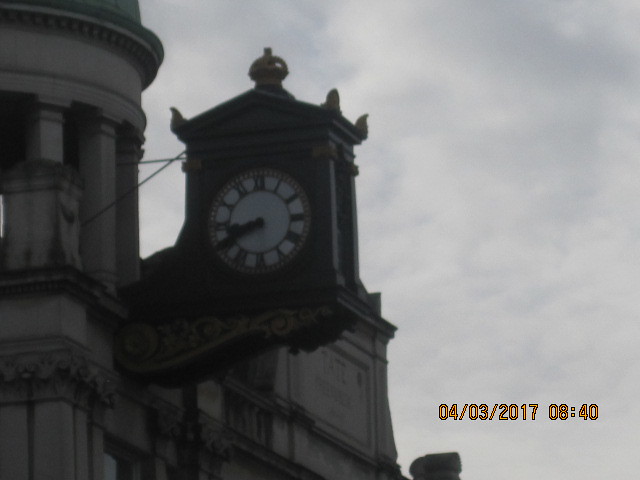This photograph, rendered in black and white, captures a clear, fair-weather day with fluffy, white clouds set against a blue sky. The focus is a large, weather-worn building made of stone and possibly cement. The building features Victorian trim and is characterized by its gray, stone facade with intricate detailing on gray pillars. Attached to the main structure is a striking clock tower. The clock tower, darker in hue compared to the building, is shaped like a house. It is crowned with a unique, ball-topped structure where each corner turns upwards. The clock itself has a white face with black Roman numerals and black hands, displaying the time as 08:40. In yellow letters at the bottom right corner of the image is the date, April 3, 2017, and the time, 08:40, further confirming the clock's reading.